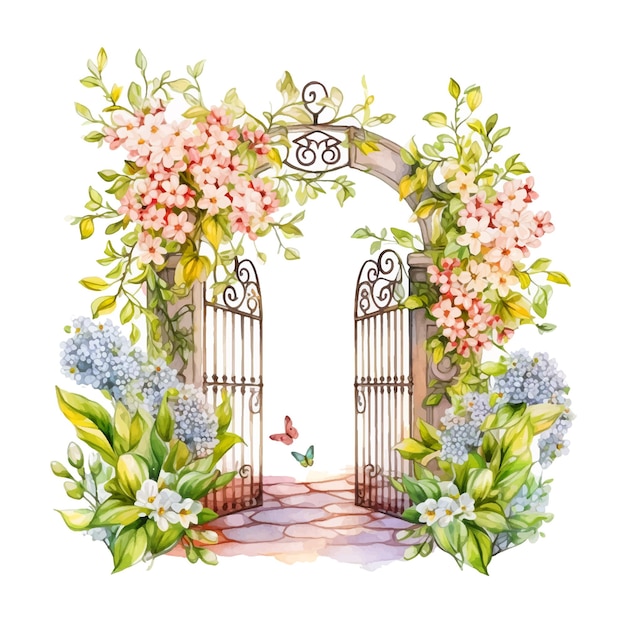This image is a richly detailed, hand-drawn colored illustration depicting a stone archway, reminiscent of a scene from a storybook. The archway, which forms an inviting entrance to what seems to be a lush garden, features an open metal gate crafted from wrought iron. The gate is slightly ajar, as if welcoming visitors. Intricate decorative metalwork is nestled at the top of the archway where a keystone would normally be found, adding an elegant touch to the structure.

The stone archway is abundantly overgrown with a variety of flowering vines that cascade down both sides to the ground. Near the top of the archway, vibrant red flowers are in full bloom, transitioning to blue flowers in the middle, and finally to white flowers at the base. Among these blossoms, there are also hints of purple and pink flowers, adding to the colorful tapestry. Two butterflies, one pink and the other green and yellow, flit gracefully through the center of the gateway, enhancing the whimsical and picturesque nature of the scene. The overall soft, watercolor style of the drawing reinforces its delicate and idyllic charm.